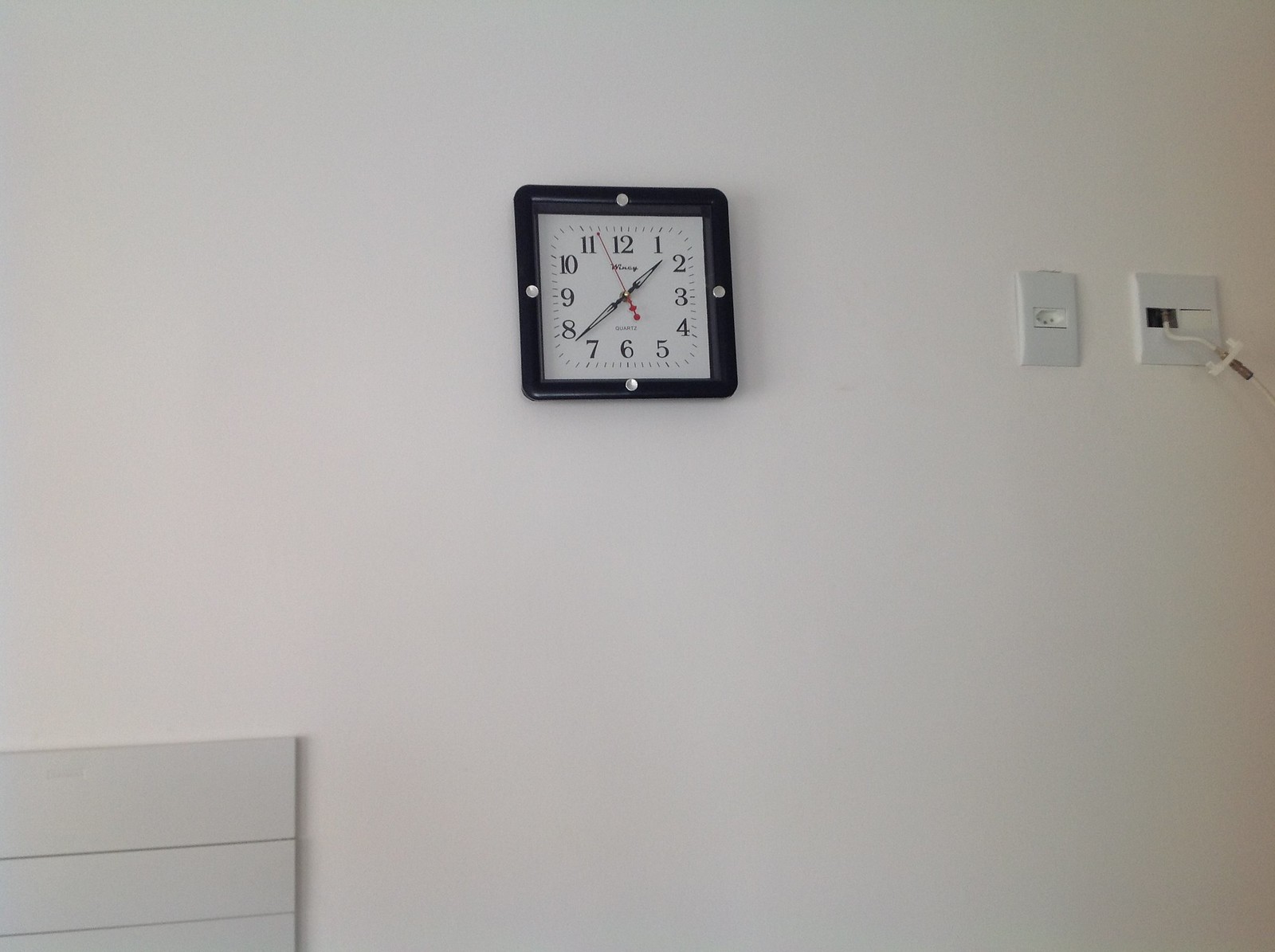This photograph captures a minimalist scene featuring a pristine white wall. In the bottom left corner of the image, a piece of a whiteboard leans against the wall, revealing its top edge and right side. Intriguingly, the whiteboard features two narrow slits running horizontally across its surface, likely where separate boards are joined.

Centrally mounted on the white wall is a square black clock with a sleek black frame. The design of the clock is accentuated by four small silver buttons, one located at each side. The clock face is equipped with traditional hour, minute, and second hands.

To the right of the clock, a white box is affixed to the wall. The front cover of this box is detached but remains hanging by a white cord, revealing its interior components. The arrangement of these elements creates a striking contrast against the muted backdrop of the white wall.